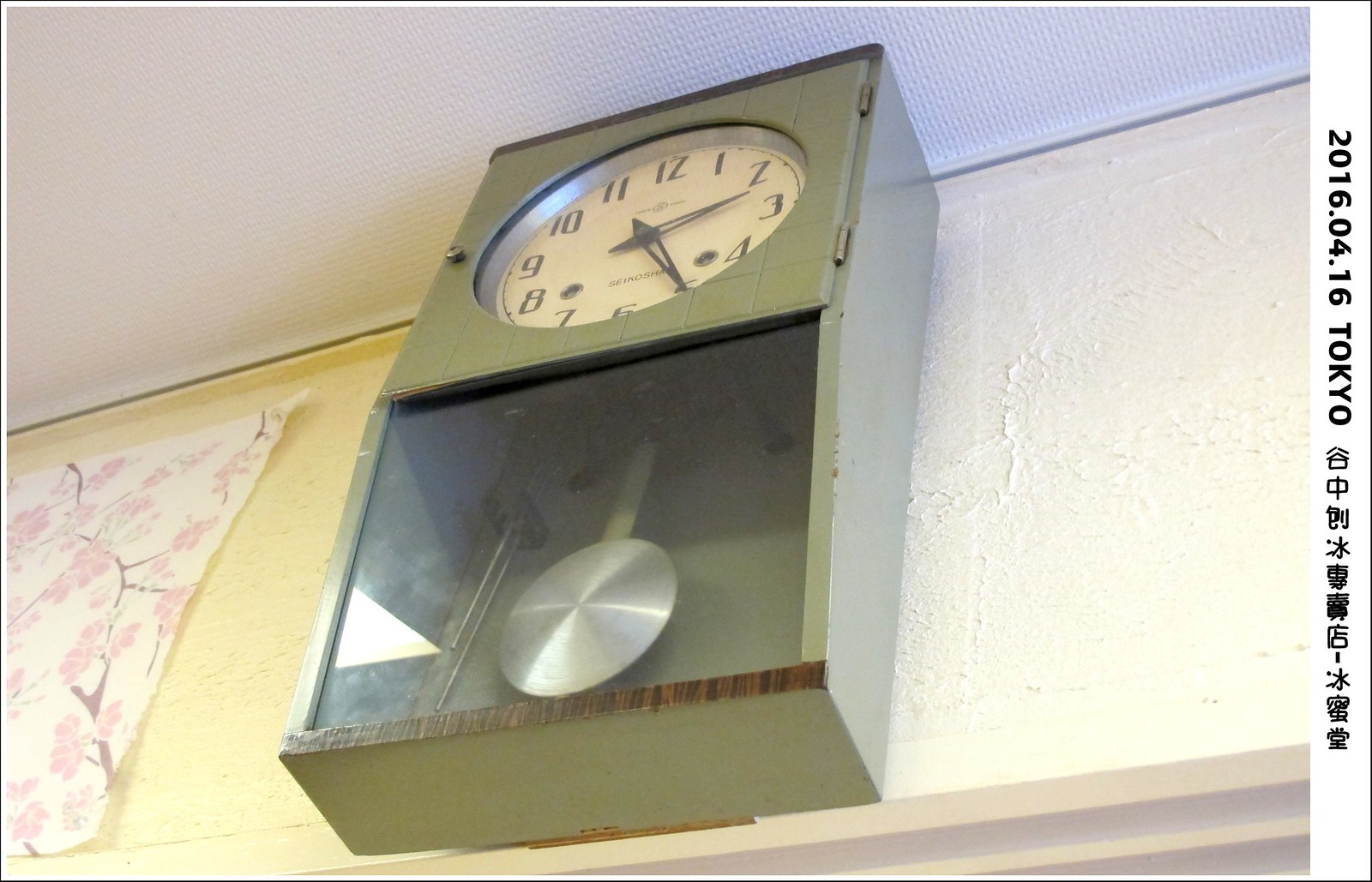The image depicts a vintage wall clock mounted on a textured off-white or yellowed plaster wall. The wall's surface is more rugged than typical drywall, suggesting it is the plaster itself that is textured. The clock is housed in an old-fashioned wooden box, painted green with a prominent grain. A small strip of dark, grainy wood is visible at the bottom front edge, hinting at its natural finish. There might be another dark wood panel at the top, but only a shadowy line is discernible.

The clock features a round face with a flat glass or plastic cover. The face has black numerals and black minute and hour hands. Left of the clock hangs a decorative sheet or paper, white with a design of small brown branches adorned with pink flowers.

Below the clock face, inside the encasement, is a silver pendulum, also set against a backdrop of black. A light brown shelf is situated directly underneath the clock. The ceiling seen in the background is painted white.

On the right edge of the image, black letters spell out "2016.04.16 Tokyo," followed by Japanese characters, indicating the date and location in Tokyo, although the specific content of the characters is unclear.